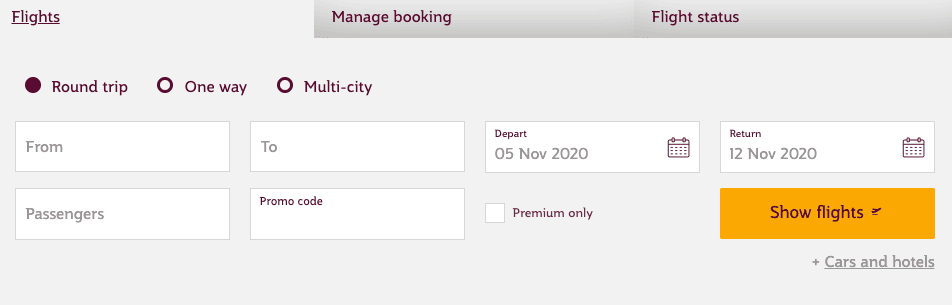The image depicts a meticulously cropped screenshot of a flight booking website interface, displayed within a small, rectangular frame. Prominently featured at the top are navigational options such as "Flights," "Manage Booking," and "Flight Status." Below, radio buttons for selecting the trip type—"Round Trip," "One Way," and "Multi-City"—are visible, with "Round Trip" actively selected.

The booking form is well-structured, including fields for "From" and "To" locations, as well as "Depart Date" and "Return Date," each accompanied by a small calendar icon for date selection. Additional fields cater to specifying the number of passengers, and there's a section for entering a promo code or opting for premium services. For added convenience, there are options to bundle car and hotel rentals with the flight booking.

The interface is visually enhanced with the "Show Flights" button, which is prominently highlighted in a vibrant red-orange hue, making it stand out as the primary call to action on the page.